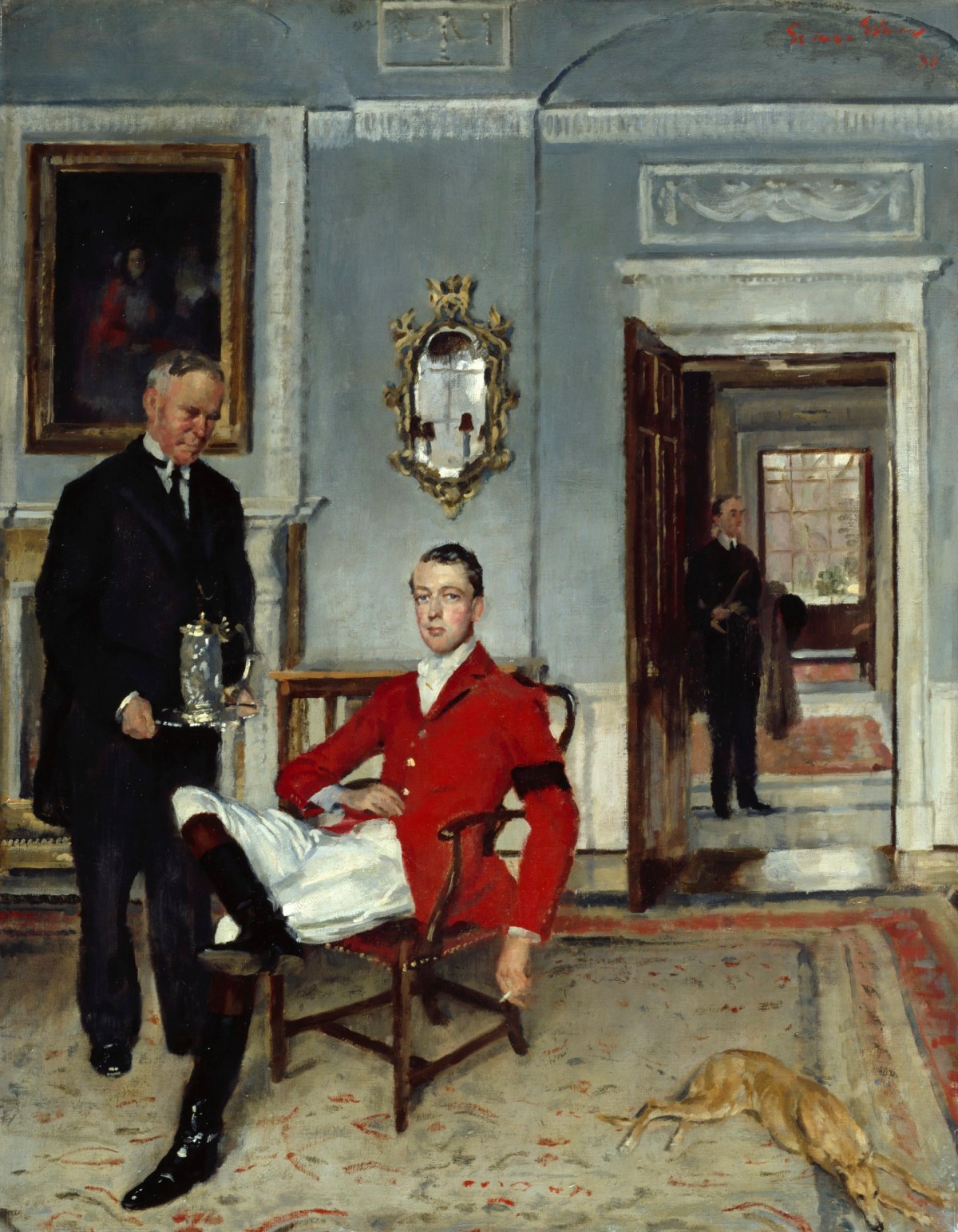This detailed painting, possibly from the 18th or 19th century, depicts a sophisticated indoor scene set in what resembles a royal palace room. Dominating the center of the composition is a young, clean-shaven white man, likely a lord or baron, seated elegantly on a chair. He is attired in a striking red blazer, white pants, a white shirt, and knee-length black boots. He holds a cigarette in his left hand, exuding an air of nonchalance. At his feet, a brown dog lies comfortably on a luxurious rug.

Nearby, a servant stands, holding a silver jug on a tray. This butler, dressed impeccably in a black coat, black pants, a black tie, a white shirt, and black shoes, appears attentive and poised to serve. The butler, an older man with very short hair, adds to the ambiance of refined service.

The room's gray walls are adorned with intricate architectural patterns and contain a vintage-era mirror with golden frames and a framed painting. To the right, an open door reveals another servant outside, clad in black clothes and holding garments, reinforcing the sense of a bustling household. There is also a second door at the far end of the room, featuring a large window that offers a glimpse of the exterior. The carefully composed elements, from the opulent decor to the sartorial elegance of the characters, contribute to an overall atmosphere of aristocratic leisure and service.